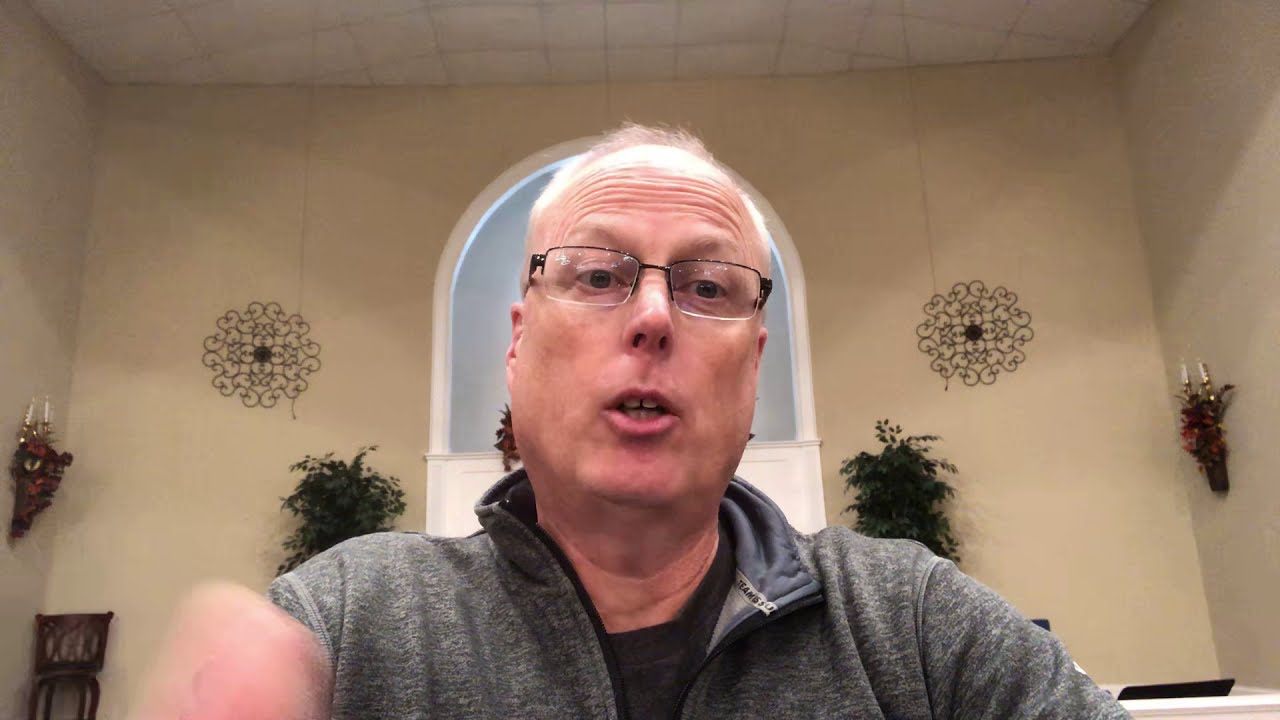A Caucasian man with light, thinning hair and wearing dark glasses stands in front of a curved window, where cream-colored walls are adorned with Spanish revival-style decorations, including intricate metal sculptures and tall plants. The man, who has very short, balding hair, is slightly looking up with his mouth slightly open, as if he is about to speak. His forehead is wrinkled, and he's wearing a gray zip-front jacket over a black shirt. In the foreground, his hand appears blurry, suggesting movement. Behind him, ornate candle sconces are mounted on the walls alongside the decorative metal artwork and greenery.